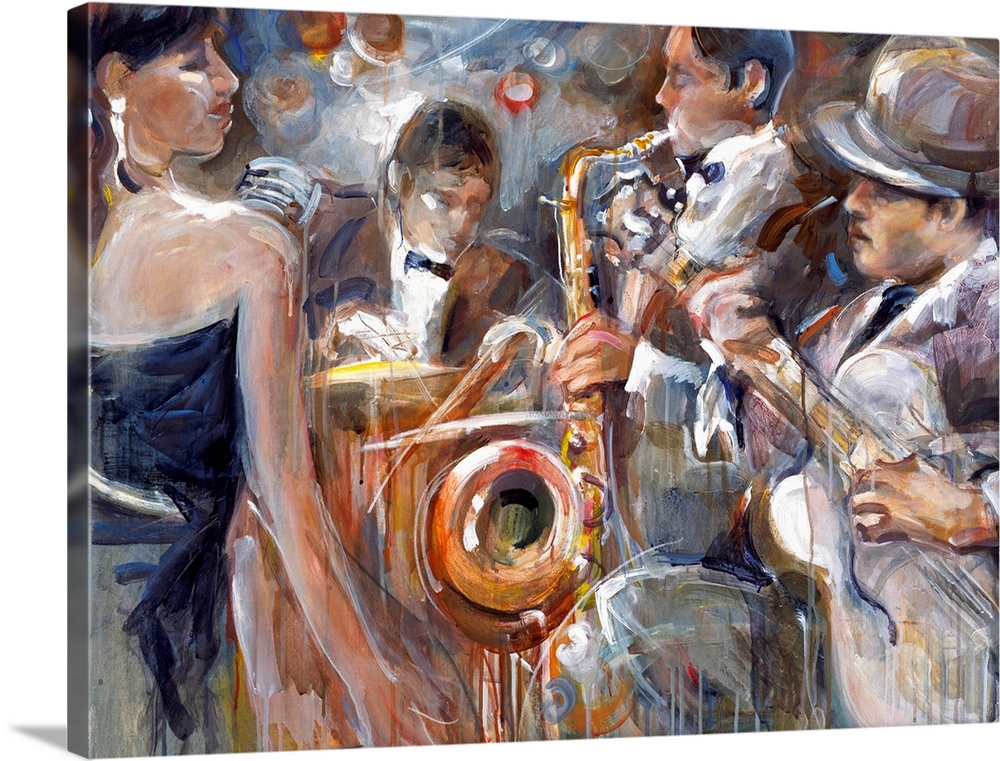In this captivating, large canvas painting, we find ourselves transported to a vibrant nightclub scene, possibly from the early 20th century. The setting exudes a lively atmosphere with a close-up focus on a jazz band, rendered in a dynamic, somewhat impressionistic style.

At the center of the composition, a gentleman in a white tuxedo and bow tie commands attention as he passionately plays a gold saxophone. His black hair contrasts sharply with the light-colored suit. To his right, another band member, dressed in a dark suit and a fedora, skillfully strums a guitar. On the left side of the painting, a sultry woman in a strapless, off-the-shoulder blue dress gazes towards her fellow musicians, her dangling earrings catching the light. She could be the singer, suggested by the presence of a gray microphone nearby.

Further enhancing the scene, another man, positioned slightly behind the central figures, wears a brown suit and stands with an air of mystery; it's not clear if he is playing an instrument. The backdrop and figures are imbued with warm nighttime hues of orange and white, lending a dreamlike quality to the overall composition. The painting's edges seamlessly extend onto the sides of the canvas, maintaining the immersive nightclub ambiance. This artwork masterfully blends distinct shapes and vivid colors, capturing the essence of a bygone era's musical vibrancy.